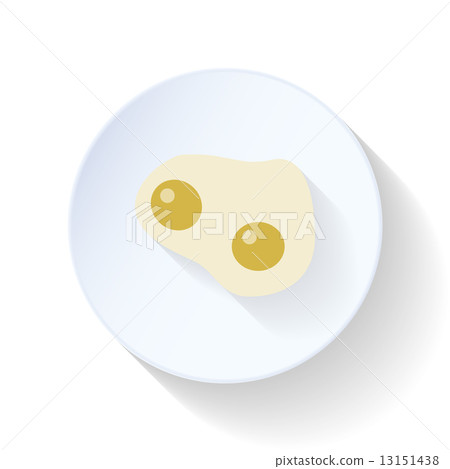This is a digital stock image featuring a cartoon-style illustration of a dinner-sized, round white plate with two fried eggs. The eggs are conjoined, sharing a single set of egg whites but featuring two distinct yolks that appear slightly brownish-yellow with a reflective dot giving them a slight sheen. The plate is devoid of any other items such as food, utensils, or napkins. Light gray text reading "PIXTA" is superimposed across the middle of the image, and the bottom right corner contains a faint watermark with the text "PIXTAstock.com-13151438." Additionally, there's a faint white line overlaying the entire image, adding to its digital artwork quality. The overall color palette is mostly white, with yellow and occasional gray tones.